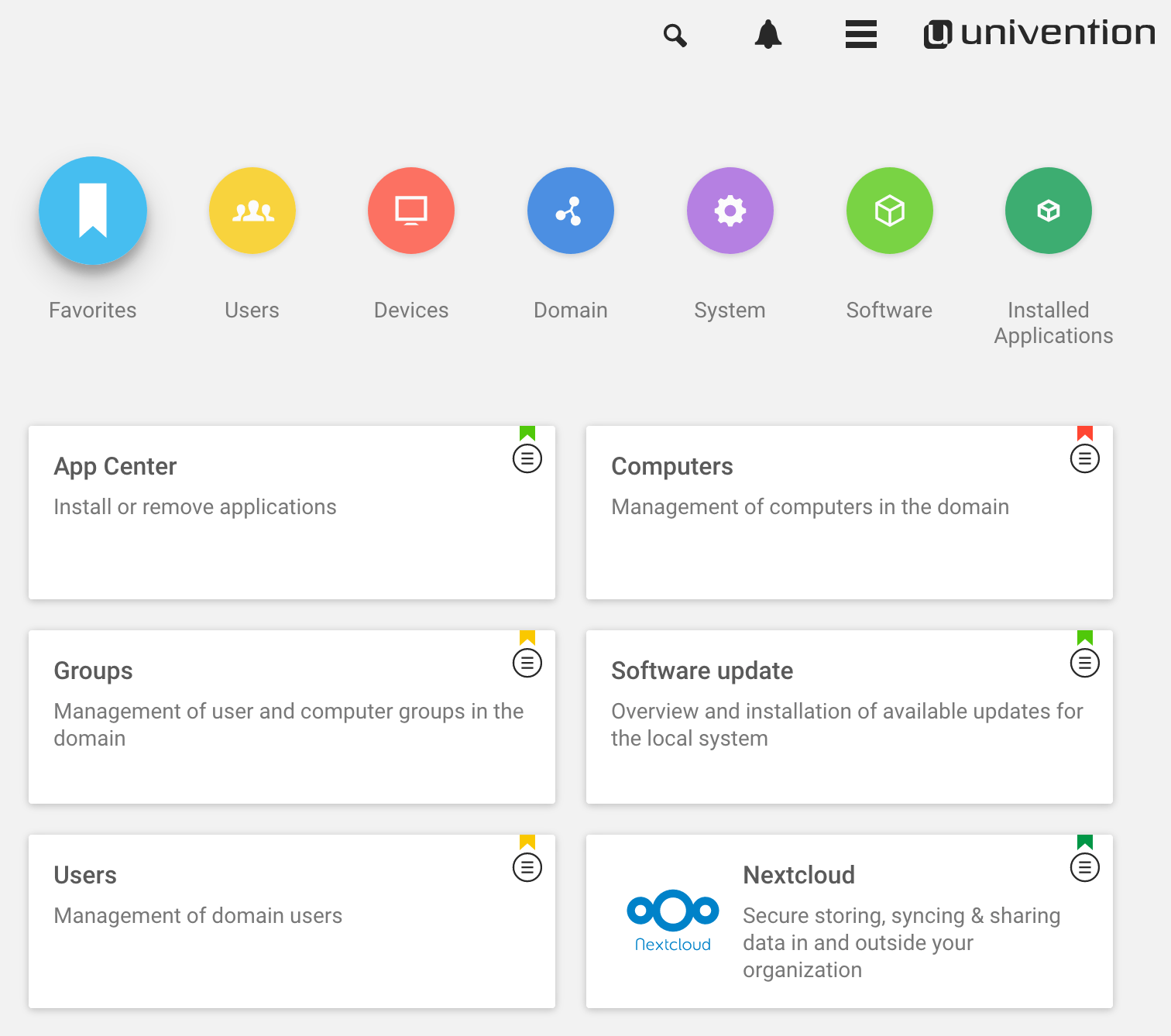The image displays a webpage belonging to Univention, identifiable by its logo in the upper right-hand corner, consisting of a capital "U" in a black box. Adjacent to the logo are three horizontal bars, an alert bell icon, and a search icon.

Prominently featured at the top of the page are seven distinct circular icons, each signaling different sections. From left to right:
1. A blue circle labeled "Favorites."
2. A gold circle labeled "Users."
3. An orange, or possibly orangey-red, circle labeled "Devices."
4. Another blue circle labeled "Domain."
5. A purple circle labeled "System."
6. A lime green circle labeled "Software."
7. A darker green circle labeled "Installed Applications."

Beneath these icons, there are six white rectangular boxes arranged in two columns. In the first column:
1. "App Center" - for installing or removing applications.
2. "Groups" - for the management of user and computer groups within the domain.
3. "Users" - for the management of domain users.

In the second column:
1. "Computers" - for managing computers within the domain.
2. "Software Update" - for overseeing and installing available updates for the local system.
3. "NextCloud" - described as a secure solution for storing, syncing, and sharing data both within and outside the organization. The NextCloud logo, consisting of one larger central circle flanked by two smaller circles, is also featured.

The layout is clean and intuitive, emphasizing ease of navigation and management within the Univention platform.